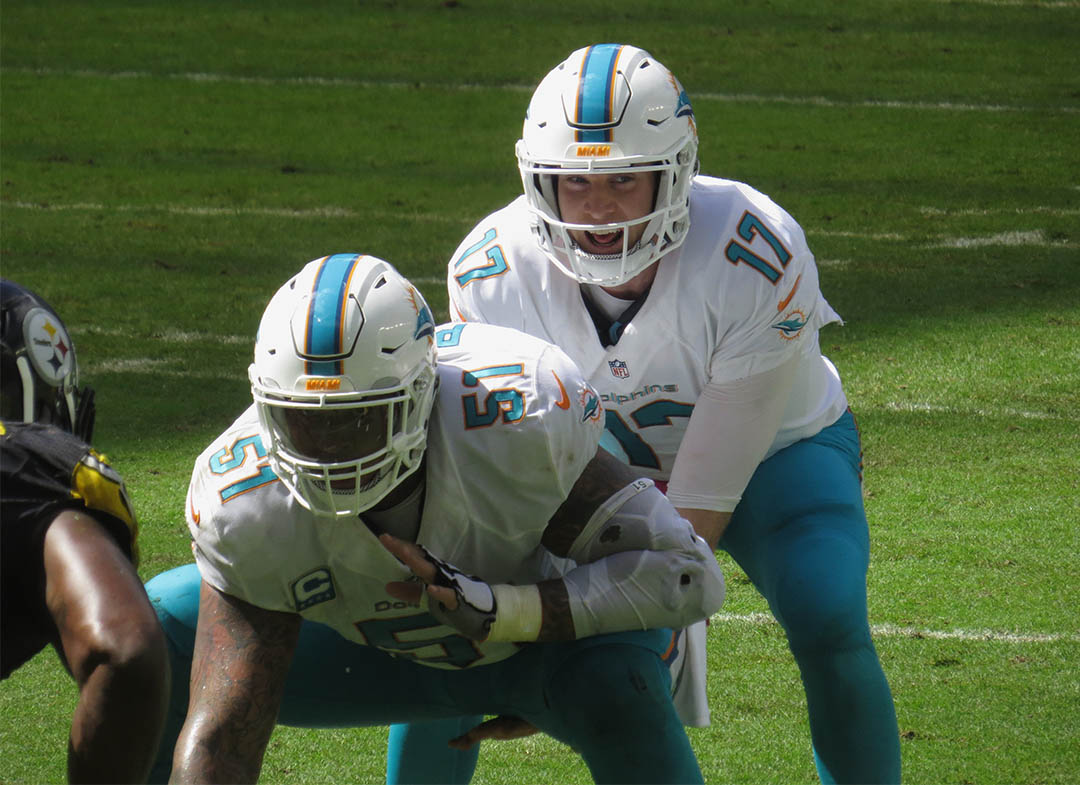In this photograph of a football game, Miami Dolphins players are prominently featured preparing for a snap. The quarterback, number 17, and the center, number 51, both stand out in their distinctive uniforms. The Dolphins are dressed in white jerseys highlighted with aquamarine accents and orange contours, complemented by aquamarine spandex. The jerseys clearly display the "Dolphins" name, and the recognizable orange Swoosh logo on the shoulders signifies their Nike sponsorship. The quarterback appears to be Caucasian, while the center is African-American, adding visual diversity to the team lineup. 

Facing them is a Pittsburgh Steeler player in a black helmet adorned with the characteristic four-color emblem, and he sports a black top with yellow accents on the shoulders. The photograph captures the tense moment just before the hike, with the quarterback under center, eyes focused, and the opposing Steeler player poised to leap into action. The backdrop is a verdant green field, bathed in sunshine that casts shadows, suggesting a pleasant fall day.